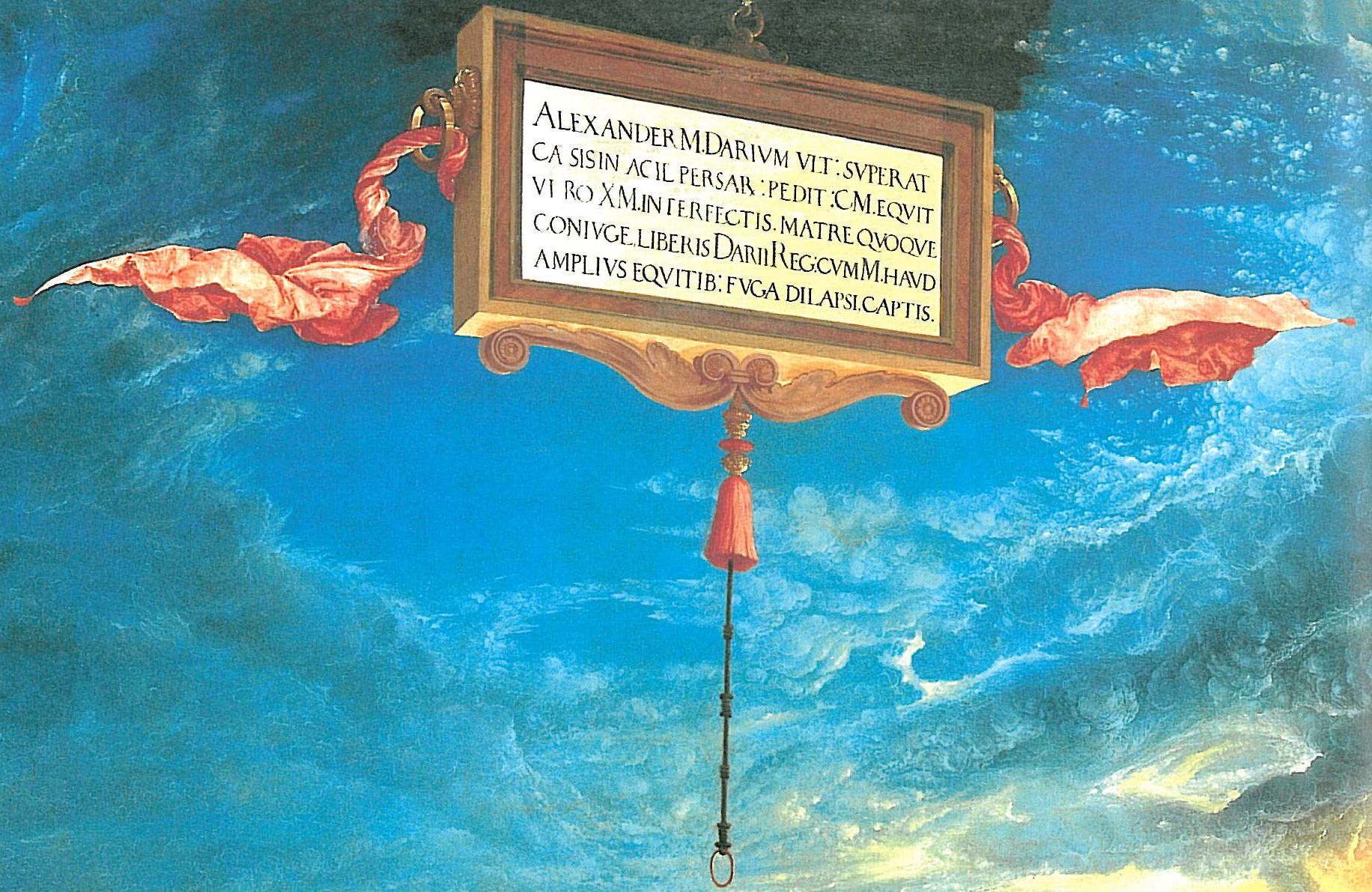This painting features a captivating and vivid background primarily composed of shades of blue and turquoise, with lighter blue areas that resemble clouds, creating a mesmerizing sky-like effect. In the bottom right corner, a patch of golden yellow adds a warm contrast to the cooler tones. 

At the center, a wooden-framed rectangular plaque appears to float in midair. The plaque contains five lines of text in black font, seemingly Old Latin, starting with the word "Alexander" and including other terms like "Darium," "Superat," and "Equivit." The white face of the plaque stands out against the richly colored background, giving it an ethereal quality.

On either side of the plaque, gold rings are attached, with red fabric banners flowing from them, adding a sense of movement to the image. Below the plaque, there is an ornate red tassel connected by a black chain to yet another gold ring, which hangs freely underneath. The entire composition creates a surreal and enigmatic scene, blending classical elements with a dreamlike atmosphere.